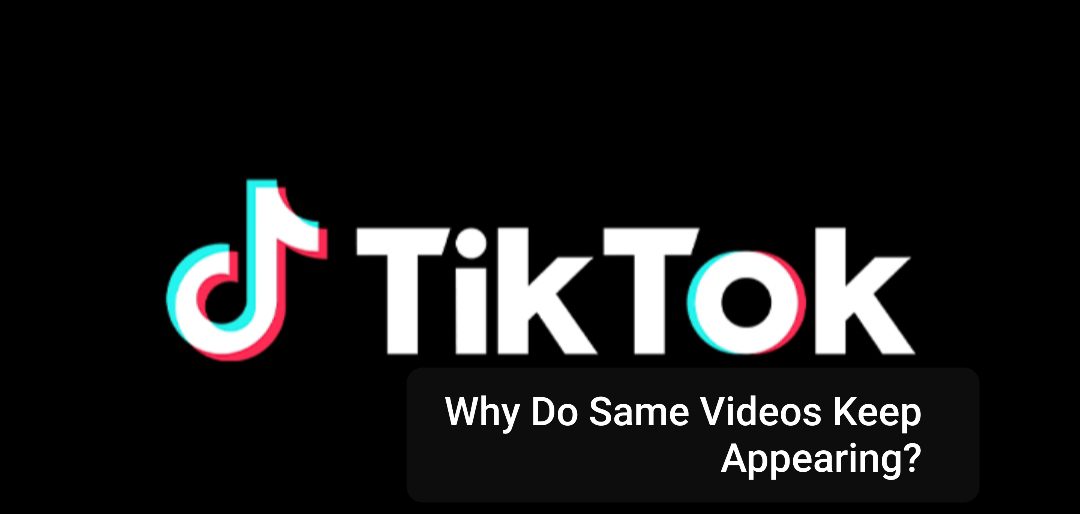This image features a simple yet striking composition. The background is a solid black rectangle, providing a stark contrast to the central logo and text. The logo, situated towards the left, resembles a partially completed music note. It's outlined with two vibrant colors – blue on its upper portion and red on the lower portion, creating a dynamic effect. 

To the right of the logo, the name "TIKTOK" is spelled out in a large, bold white font, with the letter "O" uniquely outlined in blue on the left and red on the right, echoing the color scheme of the logo.

Beneath "TIKTOK," a question is posed in smaller white font that spans three lines:
- The first line reads "WHY DO"
- The second line continues "SAME VIDEOS"
- The third line concludes with "KEEP APPEARING?"

The interrogation is accented with a question mark at the end, inviting curious contemplation. The overall minimalist design effectively draws attention to the text and logo, while the color contrast and structured layout ensure clarity and focus.